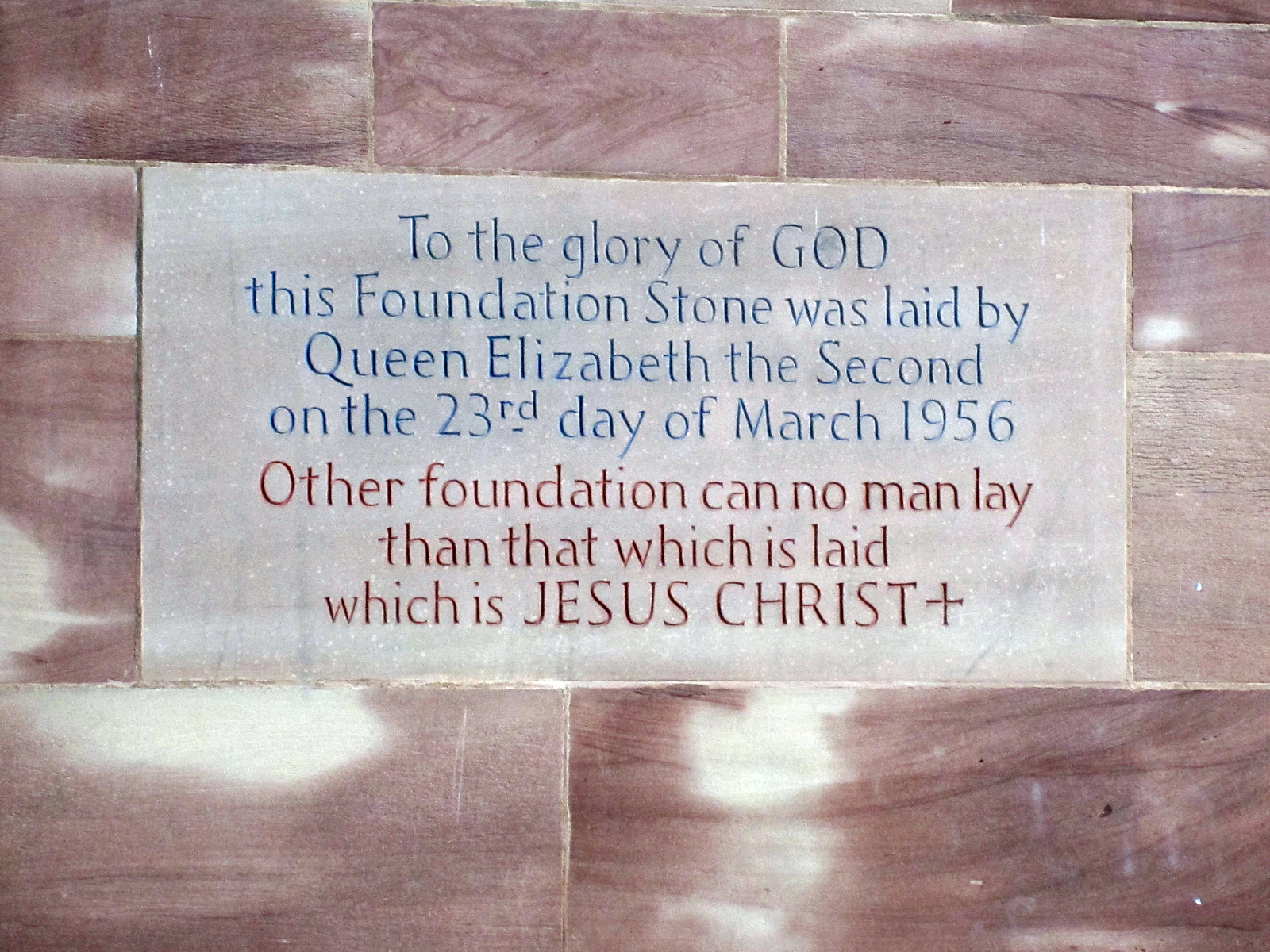The image depicts a white rectangular plaque set horizontally, featuring text that commemorates a foundation stone laid by Queen Elizabeth II on March 23, 1956. The top portion of the text, which reads "To the glory of God, this foundation stone was laid by Queen Elizabeth II on the 23rd day of March 1956," is engraved in blue. Below, in red lettering, it reads, "Other foundation can no man lay than that which is laid, which is Jesus Christ," followed by a small cross symbol next to "Jesus Christ." The plaque itself has a cement-like, marble appearance and is set against a background that appears to be wooden or possibly made of reddish granite marble cut into rectangular sections.